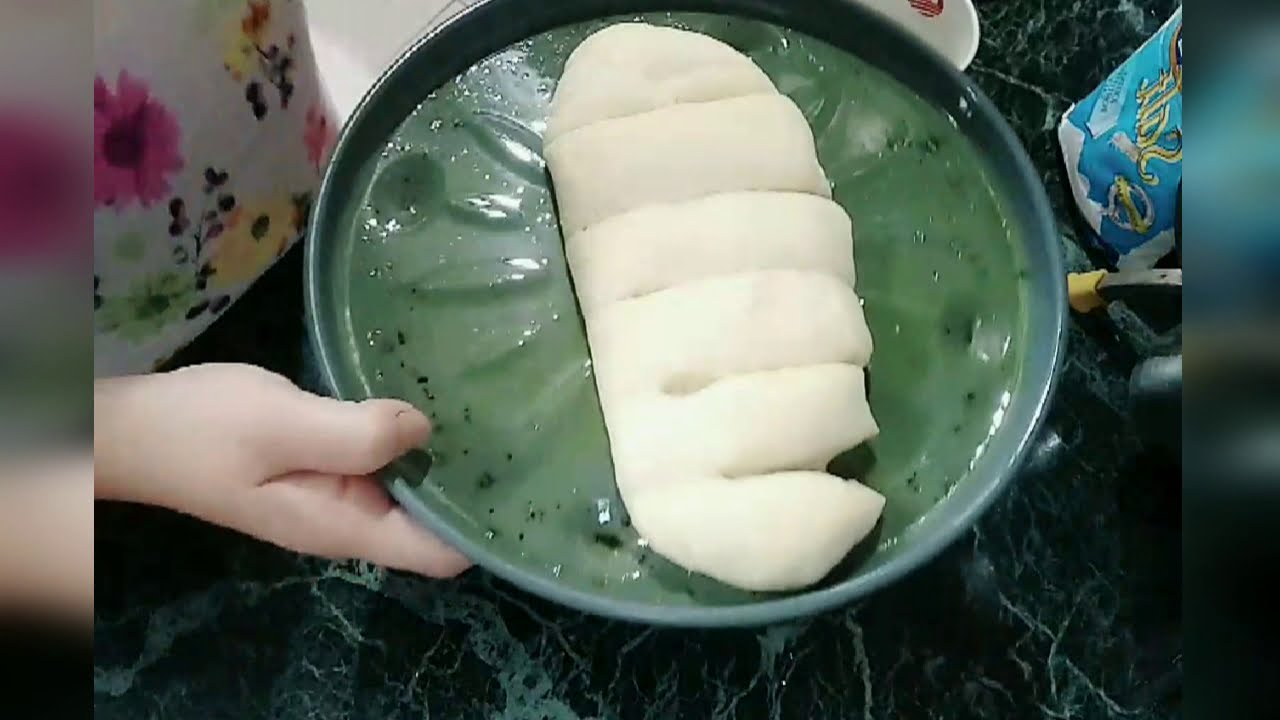In this photograph, a person with light skin is holding a circular, dark green plate that appears to be metallic. The dish showcases an unbaked loaf of bread, white in color, which has been pre-sliced horizontally. The bread dough is placed on the green bottom of the pan, with the pan's sides being silver. The person holding the plate wears a white shirt adorned with pink and yellow flowers, along with green stems and leaves, visible in the upper left corner of the image. The background features a black marble countertop with intricate patterns. To the right side of the plate, other items can be seen, including a blue object with lettering and a hint of a white bowl with some red details. The overall image retains a slightly blurry border, particularly on the outer edges.